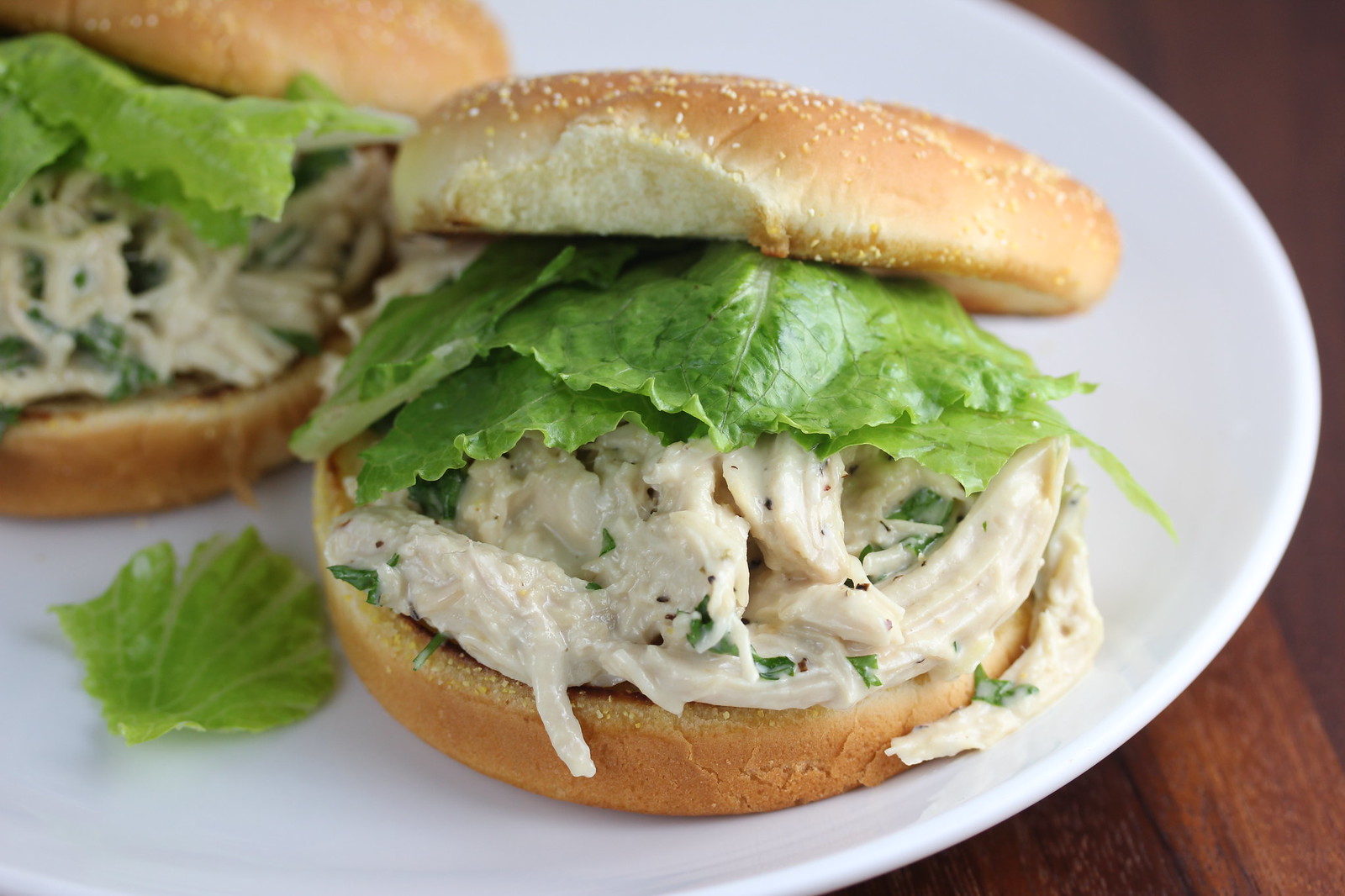The image displays two identical chicken sandwiches on a large white plate, set atop a dark brown wooden table. Each sandwich features a regular hamburger bun with sesame seeds on top and a bottom bun, encasing a layer of leafy green romaine lettuce, a filling of white meat chicken breast mixed with mayonnaise or a similar dressing, and specks of black pepper or chopped herbs. The sandwich in the foreground has its top bun slightly tilted back, revealing these detailed contents. A separate piece of romaine lettuce lies on the plate to the left of the main sandwich. The second sandwich is positioned in the upper left corner of the image, slightly blurred, yet mirroring the same ingredients and presentation.